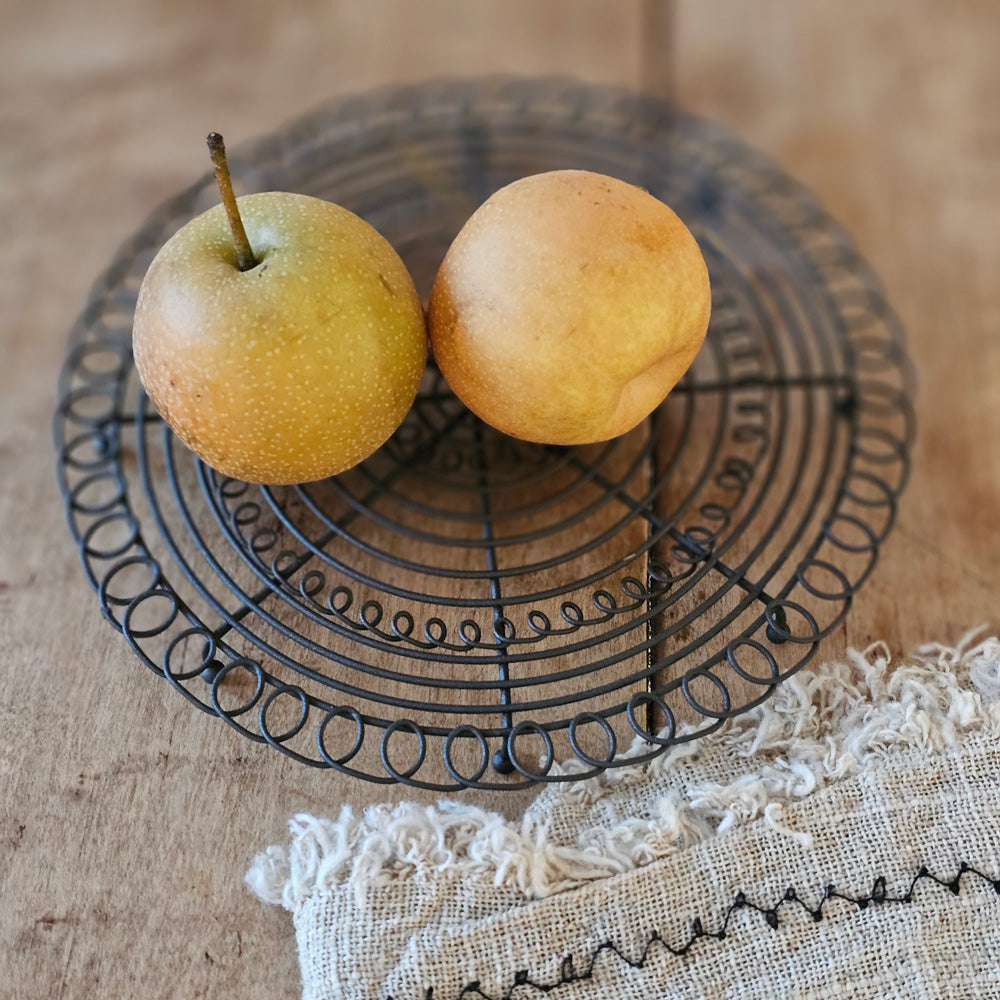The image features two yellow apples with orange undertones and white speckles. One apple, adorned with a stem, stands upright, while the other rests on its side. Both apples are placed on an ornate wire plate, intricately designed with curls and patterns along the outer rim, middle, and center. The scene is set on an unfinished wooden table composed of multiple panels, evident by the visible seams. The soft, natural light illuminating the composition hints at the photograph being taken either indoors near a window or outdoors. Adjacent to the wire plate lies a white cloth with black stitching, characterized by its visible individual strands and frayed edges, indicating a low thread count. There is no text included in the image.